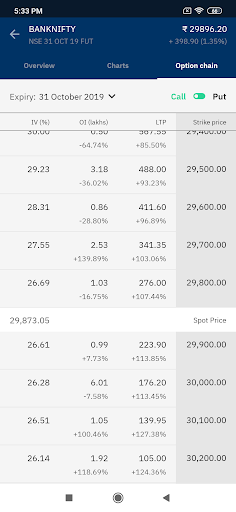This image is a detailed screenshot of a financial website's interface, specifically displaying market data for a trading platform. 

At the very top, a narrow black banner shows the current time as 5:33 PM in white text. Alongside this to the right, there are icons indicating a SIM card, Wi-Fi signal strength, and battery status.

Directly below this, a prominent blue banner features the label "BankNifty" in white text, formatted as a single word without spaces: B-A-N-K-N-I-F-T-Y. To the left of this banner, an arrow icon is visible. Below the banner, the text "NSE 31 October 19 FUT" indicates the specific market and futures data being presented.

On the right side of this section, various numerical values are displayed. The value "29,896.20" represents a significant market figure, with a corresponding increase of "+398.90" shown underneath. This increase is further clarified as a "1.35%" rise enclosed in parentheses.

Progressing downwards, the interface includes navigational options labeled "Overview," "Charts," and "Option Chain," with "Option Chain" highlighted in bold white text, suggesting it is the selected view. 

The background here is light gray, and the text "Expiry 31 October 2019" indicates the relevant expiry date for the options data. Highlighted in green, the word "Call" appears on the left side, juxtaposed against "Put" in black text on the right.

Further down, the interface lists various columns: "IV %" (Implied Volatility Percentage), "OI" (Open Interest), "LTP" (Last Traded Price), and "Strike Price," with the strike price lines set against a gray background for clarity.

At the bottom, a key figure "29,873.05" is displayed, denoted as the spot price. This is set against a gray background, providing a detailed snapshot of current market conditions.

Overall, the screenshot presents a thorough and intricate depiction of critical market metrics for users tracking financial instruments, specifically focused on the BankNifty futures expiring on October 31, 2019.